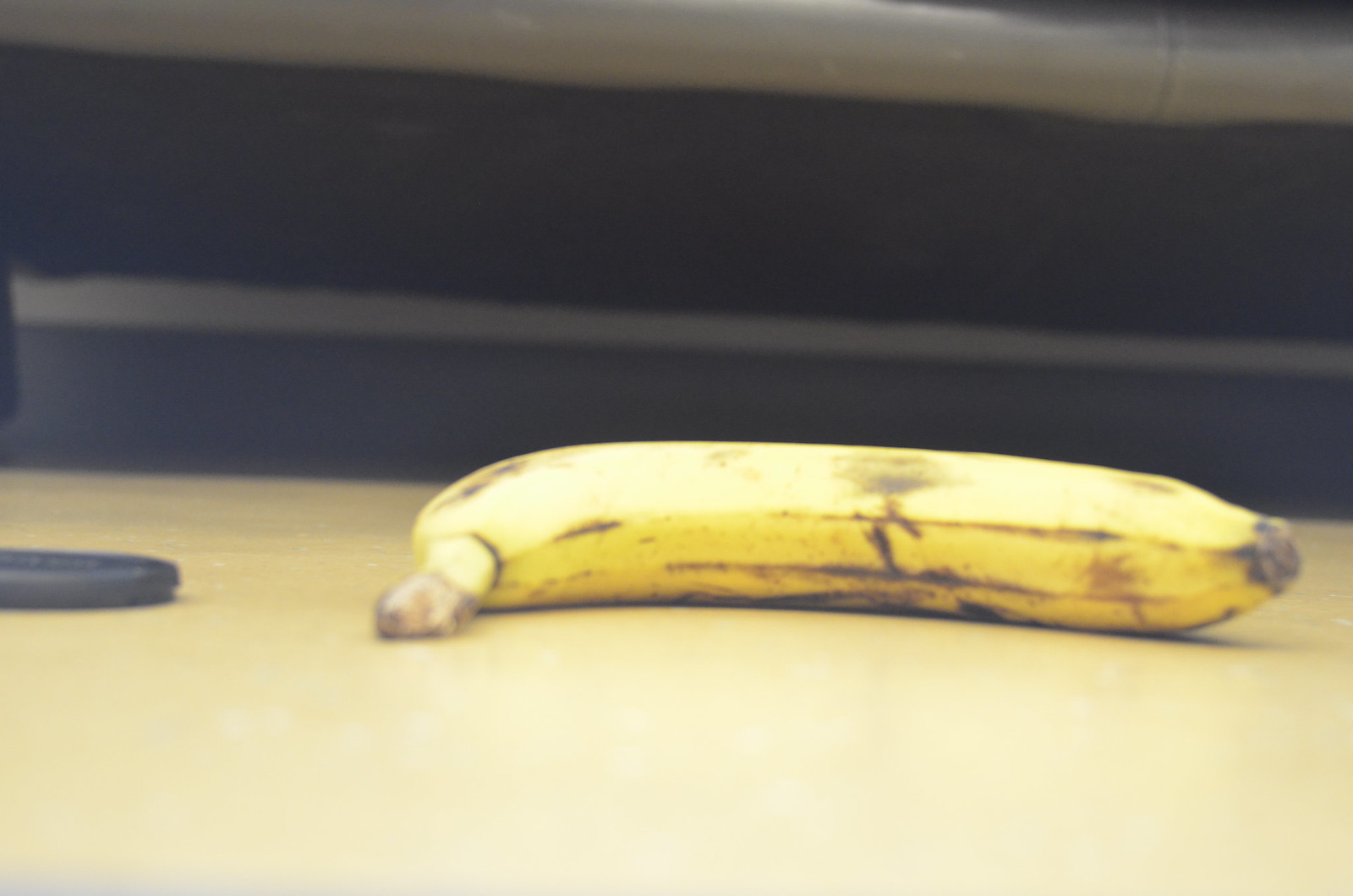In this horizontally-oriented image, a ripe banana rests on a light yellow surface resembling a table. The banana remains in its peel and displays prominent signs of ripening, with black bruises and elongated black blemishes marring its otherwise yellow skin. The top of the banana features a cut stem, tinged yellow with a dark brown edge marking the site of the cut. To the left of the banana, a small, narrow, black object of man-made origin lies parallel to the fruit; it seems to be crafted from plastic. The background reveals a wide horizontal black stripe above a broad, grayish-dark band, separated by a thin white line. At the very top edge of the image, a cylindrical metallic line, shiny and silver like a piece of polished pipe, runs horizontally.